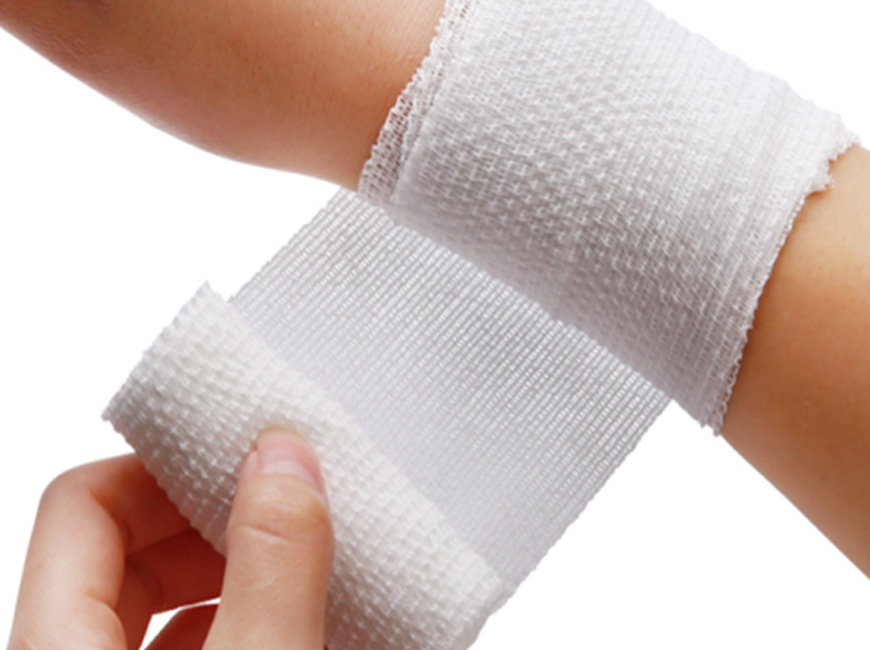This detailed photographic image, set indoors and in landscape orientation, captures a person's left wrist being wrapped with a white knit bandage. The photograph is devoid of any text and emphasizes the hands involved in the action. The bare, unpolished fingernails suggest the hands could belong to a person of any gender, possibly a white woman, although this is speculative. 

The bandaged wrist enters the image from the top left corner and extends almost to the middle of the right side, showcasing layers of white bandage already in place. The wrapping appears uneven, with some edges slightly ragged. Below, in the bottom left corner, the person's other hand – primarily visible are the thumb and partial fingers – holds and stretches the bandage, methodically applying it to the wrist. The texture of the knit fabric, about two and a half inches wide, is pronounced, showing raised rows. The action suggests a careful, though not perfectly neat, procedure of bandaging the wrist.